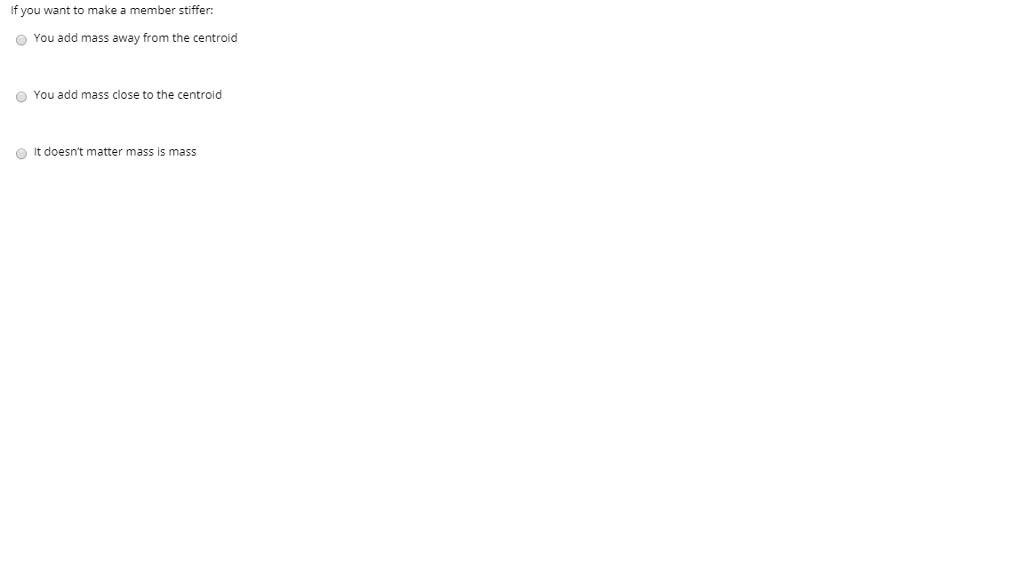A screenshot of an online engineering or physics test is displayed. The screenshot is predominantly white with a singular line of small black text positioned toward the upper left corner. The text reads, "If you want to make a member stiffer;" followed by a list of three multiple-choice options. None of the three radio button options are selected. The options are: 

1. "Add mass away from the centroid"
2. "Add mass close to the centroid"
3. "It doesn't matter, mass is mass"

The choices are evenly spaced but closely packed near the question text. The rest of the page appears empty, suggesting that this could be part of a larger interface that is not fully captured in the screenshot.